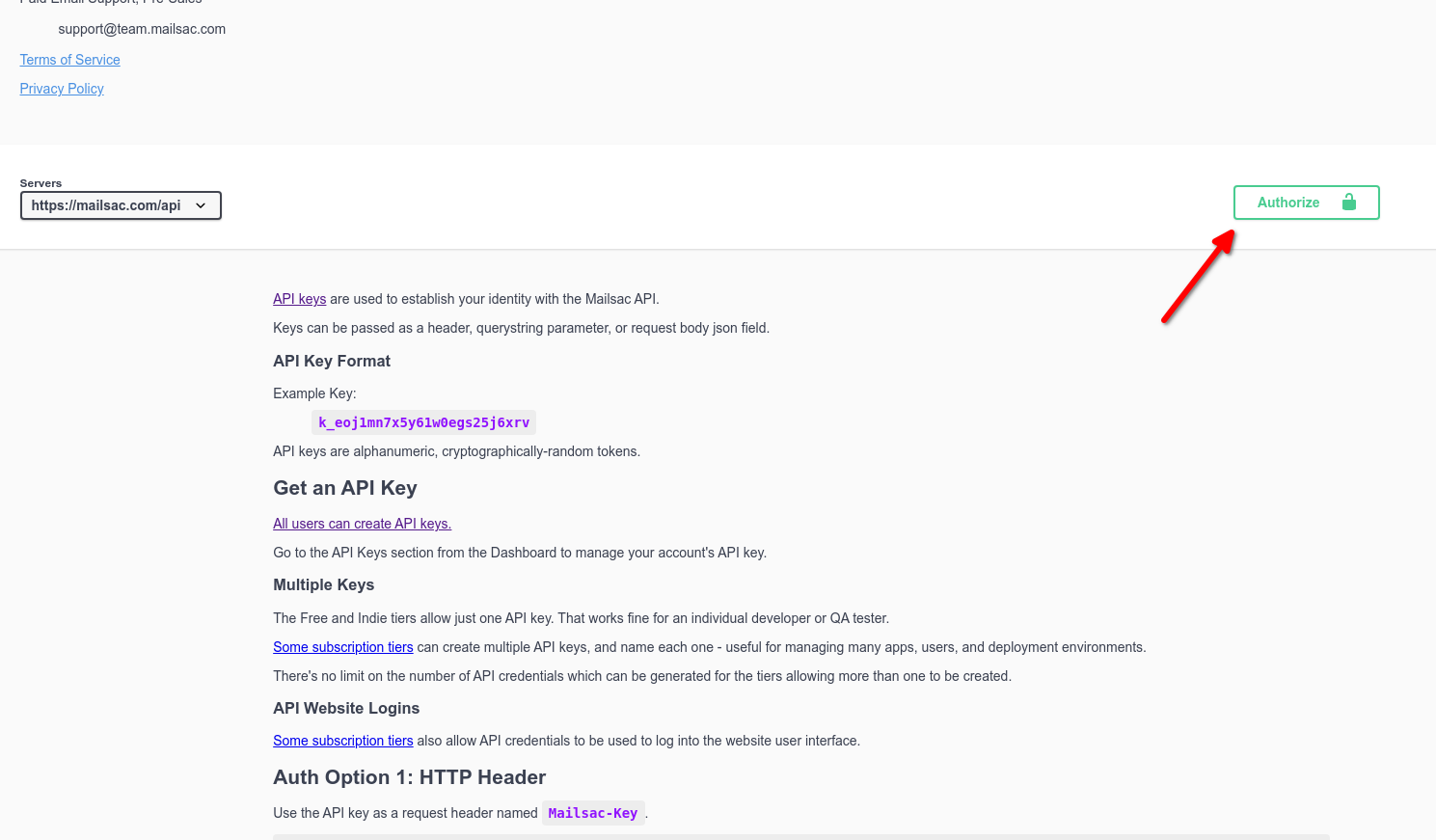In the image, a white background serves as the canvas. Dominating the top section is a prominent blue box, partially obscured by a cut-off blueprint in the top-left corner, hinting at some detailed schematics. Within this blue box, there's a lightly visible supply line of text linking to "support@team.something.com," flanked by underlined terms such as "Terms of Service" and "Privacy Policy" in blue.

Beneath the blue box lies a white box containing the word "Services," immediately capturing the viewer's attention. Directly below this, a URL "httpsmailsack.com/API" stands out, framed in a blue box. To its right, the word "Authorized" is notable, accented with a blue lock icon adjacent to it, while a red arrow points upward toward the "Authorized" label, emphasizing its importance.

Further down, the background transitions into another blue section, elaborating on API details. Text highlights include "API" and "API Key Format," followed by an example and instructions on how to obtain an API key. Additional information outlines the use of multiple keys and API website logins. There are references to "substitution terms," which are also in blue and underlined for emphasis.

Toward the end, the text delves into authentication options, specifically mentioning "Option 1 HTTP Header," and culminating with a few purple letters, adding a distinct splash of color amidst the mostly blue and white palette.